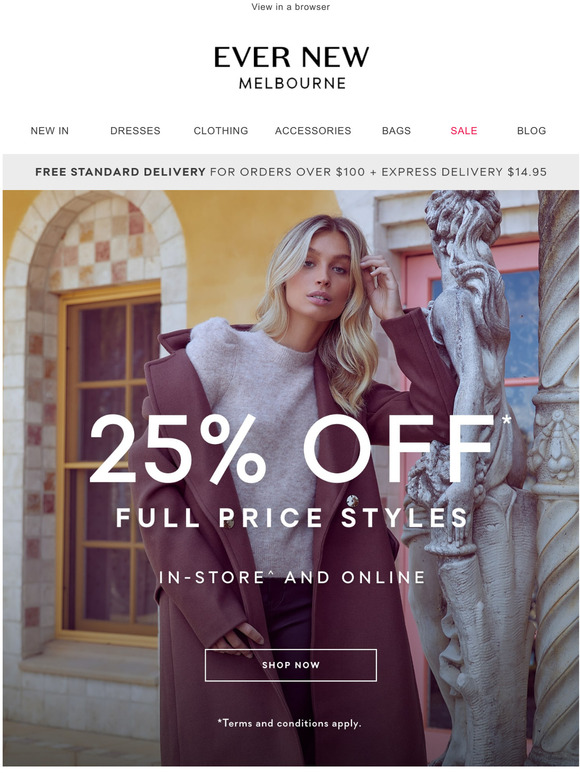The image is a screenshot of the Evernew shopping site. At the top, centered in black text, is the name "Evernew," with "Melbourne" positioned just beneath it. Below this heading, a navigation menu spans from left to right with categories listed as "New In," "Dresses," "Clothing," "Accessories," and "Bags." The word "Sale" appears in red type, followed by "Blog." A gray border runs horizontally across the page below the menu, with the bold text proclaiming "Free Standard Delivery for orders over $100, express delivery $14.95."

The main content of the image shows a photograph filling the rest of the screen. The background features a yellow-painted building with a large window on the left, which has an arch and yellow panes. Standing in front of the building is a young Caucasian woman with long, wavy blonde hair. She is dressed in a gray shirt and layered with a long brown coat. Overlaying the image of the woman, bold text reads, "25% off full-price styles, in-store and online," followed by a rectangular button that says "Shop Now" and a note beneath it stating, "Terms and Conditions Apply." To the right of the woman, she is leaning against a gray, intricately carved statue of what appears to be a person.